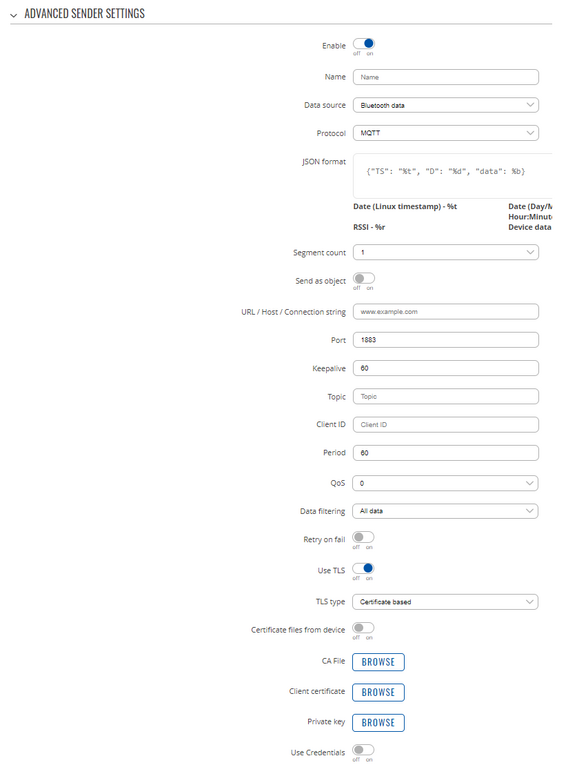The image depicts a detailed settings page related to advanced sender configurations. In the top left corner, there is a section labeled "Advanced Sender Settings". The options available include:

- **Enable**: Toggle to turn the sender settings on or off.
- **Name**: Field to specify the sender's name.
- **Data Source**: Choose between various data sources such as Bluetooth data.
- **Protocol**: Options include MQTT, with the following settings:
  - **JSON Format**
  - **Date** and **Linux Timestamp**
  - **RSSI** (Received Signal Strength Indicator)
  - **Segment Count**
  - **Sender's Object**
  - **URL or Host or Connection String**
  - **Port**: Default set to 1883
  - **Keepalive**: Interval set to 60
  - **Topic**
  - **Client ID**
  - **Period**
  - **Quality of Service (QS)**
  - **Data Filtering**
  - **Retry on Fail**
  - **Use TLS**: Toggle for enabling TLS, with type options including certificate-based secure connection
- **TLS Type**:
  - **Certificate-Based**: Requires certificate files
  - **CA File**: Option to browse and upload a CA file
  - **Client Certificate**: Option to browse and upload the client certificate
  - **Private Key**: Option to browse and upload the private key
  - **Use Credentials**: Toggle for enabling credential-based security, set to off by default
- **Sender's Object**: Setting also has an enable/disable toggle, currently off
- **Enable**: This toggle has been switched on.